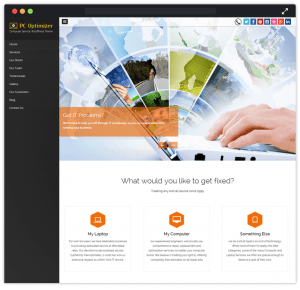In this image, the edges are bordered by a black frame. In the upper left corner, there exists an arrangement of red, yellow, and green lights along with a small dot and some red text. There are several light gray subtitles scattered across the area. Dominating the central portion of the image is a large white box. At the top of this box, there is a small black square. On the right side of the box, there are several smaller squares, presumably icons for social media platforms like Facebook and Twitter.

Inside the central white area, there's an intriguing graphic resembling a semi-circle, partitioned like a pie chart, with various colors and images within the slices—blue and green sections, alongside a red square featuring white text. To the right of this graphic, a person's hands are shown typing on a keyboard.

Below this segment, a white box contains the text "What would you like to get fixed?" Beneath this, there are three smaller orange boxes, each emblazoned with distinct images.